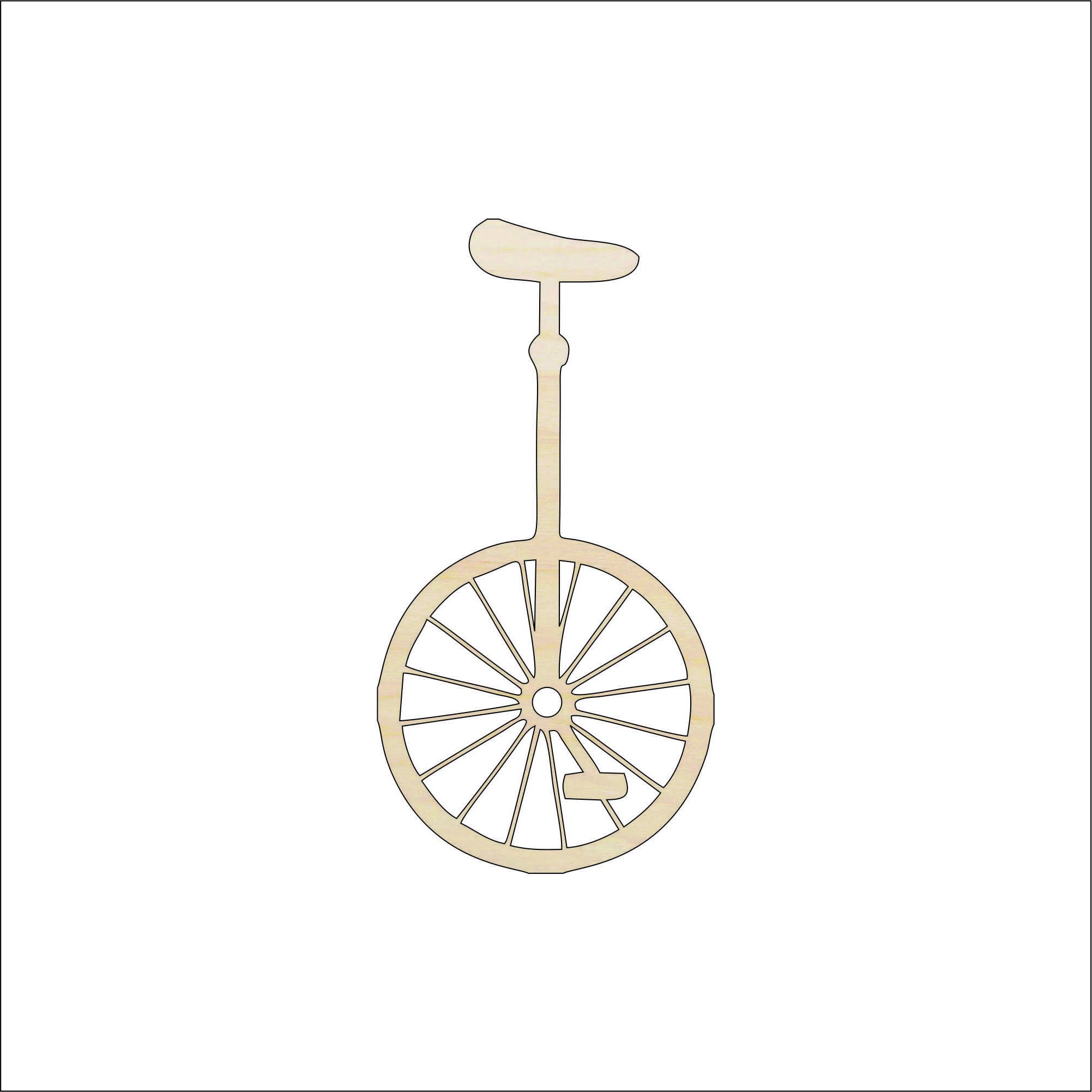The image shows a detailed drawing of a unicycle centered against a white background. This unicycle illustration is primarily an outline with a light beige or peach-colored hue. Starting from the top, the drawing features the seat of the unicycle, which extends downwards in a straight line before slightly curving and then continuing straight to form the wheel. The wheel is described with an expanded shape, resembling a slice of an orange, and clearly shows the axle and center of the wheel. Additionally, one pedal is visible. The drawing is set within a thin black border, and the overall presentation of the image is clear and bright with no other objects or text present.